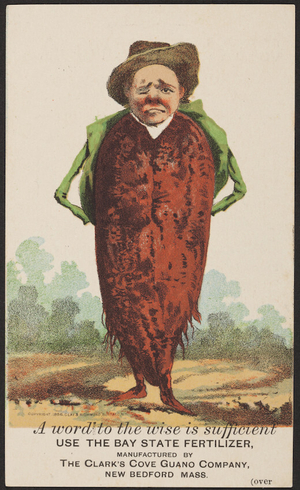The poster features a tall and slender arthropomorphic vegetable figure, resembling a human with the features of a potato or radish, set against a predominantly gray and cream background with watercolor accents of trees and grass. The figure is dressed in a reddish-brown cloak or dress with a small green jacket, contrasting his tiny red feet and thin arms. His expression is forlorn, marked by one eye half-closed and the other open, rosy cheeks, and a frown, topped with a rickety, out-of-shape cowboy hat. Below the artwork, in black italic text, reads "A word to the wise is sufficient," followed by bold all-caps instructions: "USE THE BAY STATE FERTILIZER MANUFACTURED BY THE CLARK'S COVE GUANO COMPANY, NEW BEDFORD, MASSACHUSETTS." The poster, set in a portrait layout framed by a black border, subtly suggests that the vegetable figure's discontent is due to not using the advertised fertilizer. An additional note in the lower right corner states "(over)" indicating more information on the reverse.